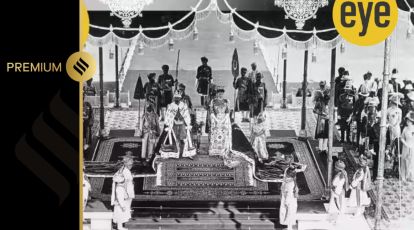The image is a horizontally aligned rectangular picture, predominantly black and white, with distinct detailed features enhancing its regal theme. On the left side, there's a thick solid black border with the word "PREMIUM" printed in gold uppercase letters. A vertical gold line separates this border from the rest of the image. The scene within the image appears to depict a coronation ceremony, centered around a king and queen seated on a platform. The king, sitting to the left, and the queen, on the right, are adorned in heavy ornate robes, and are surrounded by people, likely guards, holding flags and standing in uniforms. The upper right corner of the image features a small gold circle, with the word "i" printed in lowercase black letters. Above the central figures, an ornate canopy with fringe hangs down, adding to the grandeur of the ceremony. Despite the clarity of the words and other design elements, the overall image of the people is notably blurry, giving an impressionistic feel to the historical event depicted.